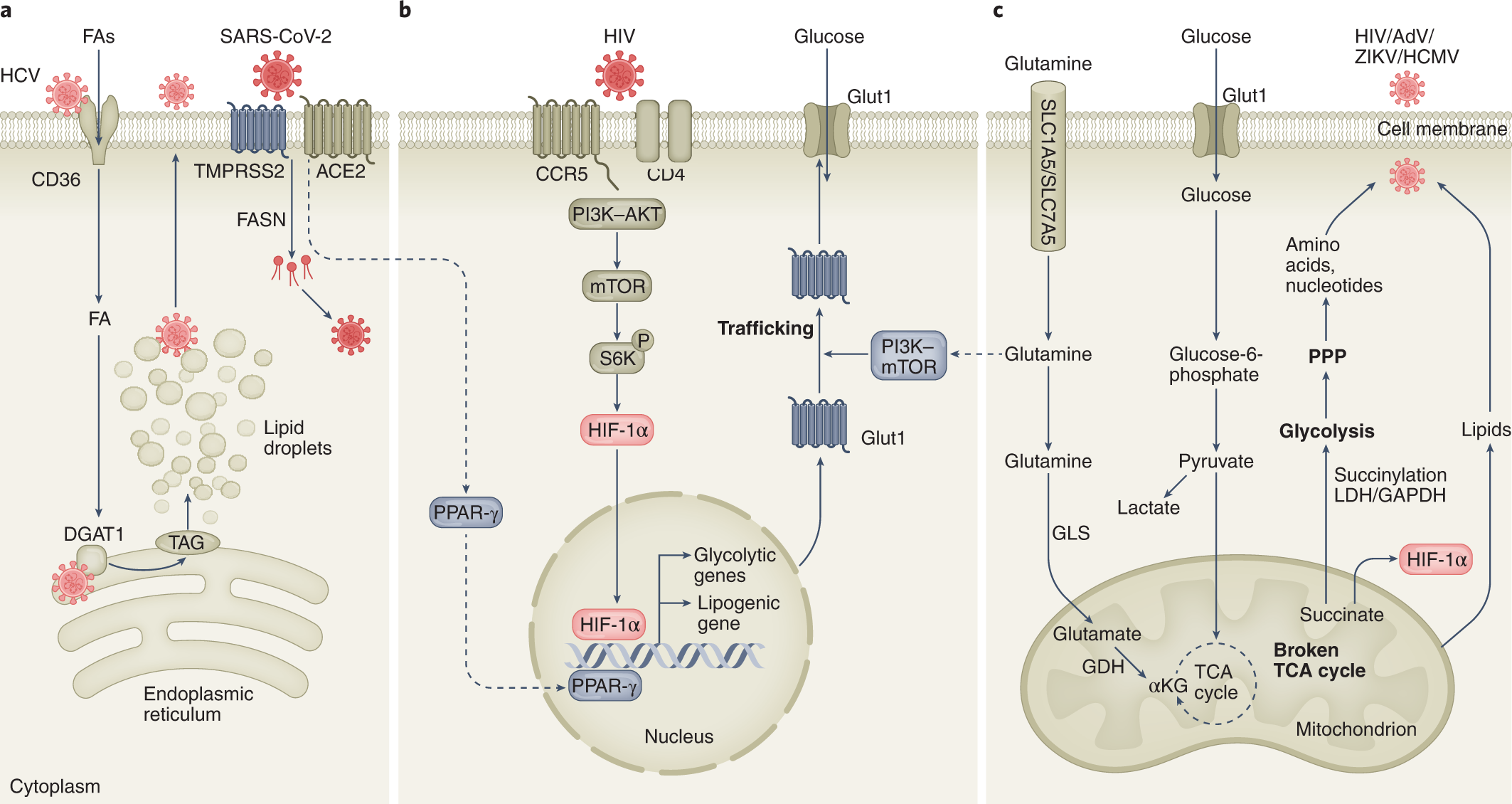This composite image features three interconnected diagrams labeled A, B, and C, each detailing the biochemical processes associated with different viruses on human cells, set against a beige background. Diagram A illustrates the SARS-CoV-2 virus's interaction with cellular components, showing arrows depicting its entry and exit pathways. It features spherical elements labeled with terms such as "endoplasmic reticulum," "cytoplasm," and specific abbreviations indicating various stages of viral trafficking. Diagram B focuses on HIV and glucose metabolism, highlighted by central figures like "glycolytic genes" and "lipogenic gene." It illustrates metabolic processes with arrows indicating directional flow and includes other labels like "nucleus" and elements of cellular metabolism. Diagram C presents biochemical pathways involving glutamine, with arrows highlighting its role in energy production and synthesis pathways, labeled with "SLC1A5," "SLC7A5," and various metabolic cycles such as the "TCA cycle," alongside breakdowns of amino acids, nucleotides, and lipids. The diagram also mentions interactions with other viruses, like HIV, ZikV, and HCMV, providing a comprehensive overview of viral impact on cellular structures and functions.